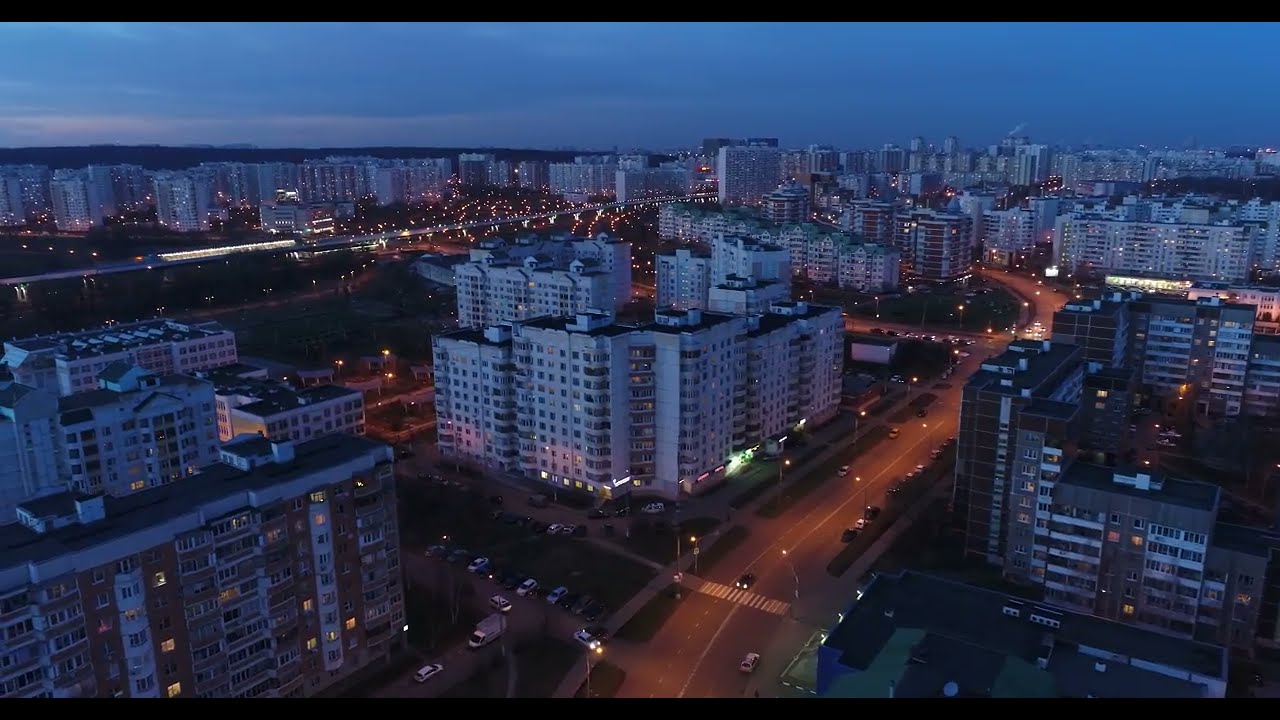This is a drone shot capturing an expansive urban landscape at the onset of night, likely 20 to 30 minutes after sunset. The scene is bathed in a purply tinge with a dark, cloud-covered sky taking up the top eighth of the image. The sky is almost black, contributing to the overall twilight ambiance. The city comprises numerous white, modern apartment buildings, uniformly lit with twinkling lights that enhance the city's clean appearance. These structures range from 6 to 15 stories, with a few taller ones reaching upwards. The buildings are largely angular, with some slight variations in shape. 

A significant reddish boulevard runs from the center-bottom of the photo, curving left towards the background, intersecting various brightly lit streets and highways, particularly noticeable in the top left corner with buildings stretching behind. The foreground reveals a densely packed arrangement of buildings and roads, leaving minimal visible green spaces, which are barely discernible due to the darkness. The overall impression is of a densely populated and meticulously organized urban setting, punctuated by the glow of streetlights and the illuminated windows of numerous high-rise buildings.